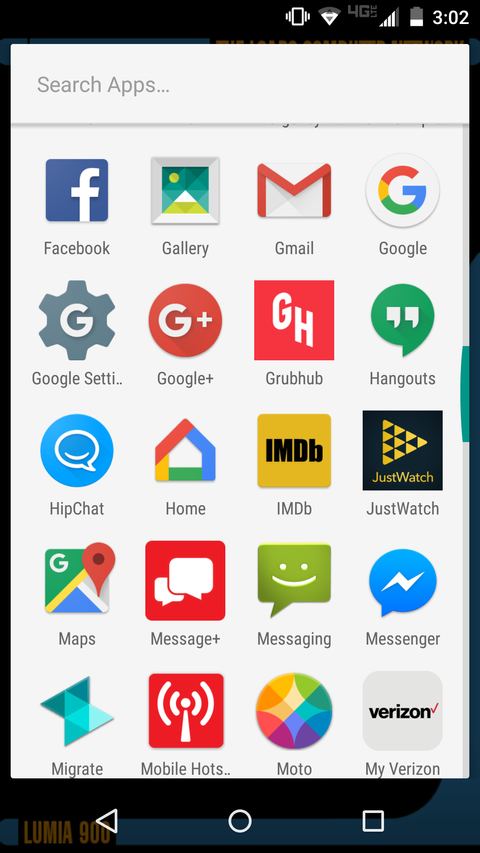A screenshot of a smartphone display showing a collection of application icons under the "Search Apps" page. The phone shows a 4-bar LTE signal indicator with 25% battery remaining. The status bar also indicates an active Wi-Fi connection with a weak signal. The displayed applications include:

- Facebook
- Gallery
- Gmail
- Google
- Google Settings
- Google Plus (discontinued)
- Grubhub (discontinued)
- Hangouts (discontinued)
- HipChat
- Home
- IMDB
- Chestwatch
- Maps
- Message Plus
- Messaging
- Messenger
- Migrate
- Mobile Hotspot
- Mobile Hots
- Moto
- Verizon

At the top of the screen, there is a search bar labeled "Search Apps." The navigation bar at the bottom of the screen includes the back, home, and menu buttons. Notably, the menu button displays "Lumia 900," which might be the model number of the phone. The background is white, and the app icons are colorful, providing a vivid contrast.